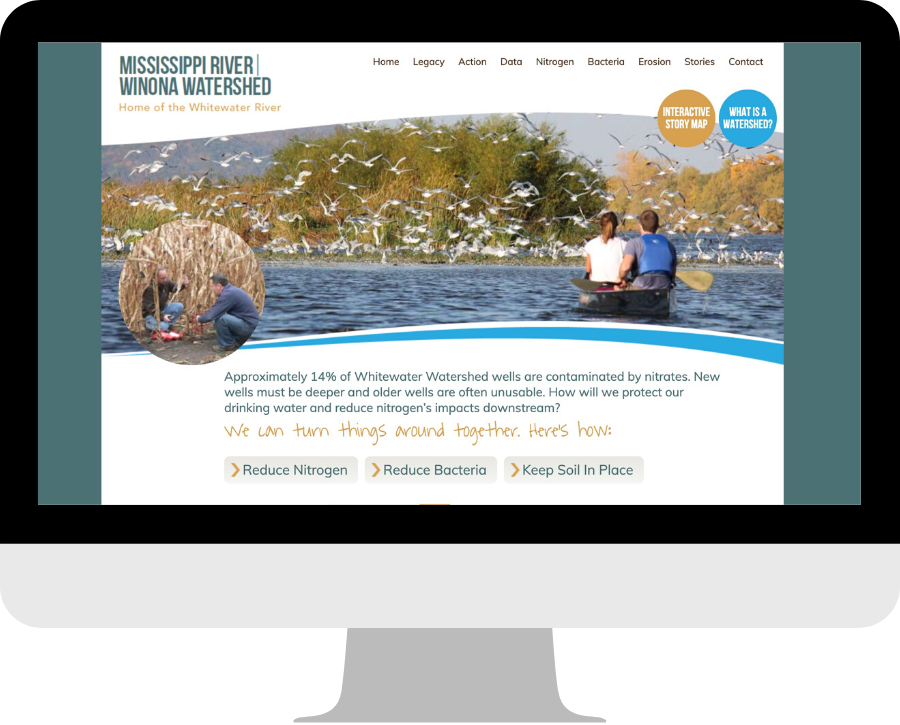This image is a graphic mock-up of a computer desktop monitor displaying a website for the Mississippi River Winona Watershed. The monitor is a simplistic, clip-art style flat-screen. The website features a white background with "MISSISSIPPI RIVER WINONA WATERSHED" prominently displayed in large blue capital letters at the top left. Beneath this header, in smaller orange letters, is the tagline, "Home of the Whitewater River."

Towards the top right of the screen, there is a navigation menu with categories listed in small black letters: Home, Legacy, Action, Data, Nitrogen, Bacteria, Erosion, Stories, and Contact.

The main content area of the page features a large rectangular photo that gently waves at the top and dips slightly down on the right. This image shows two people in a kayak on a river, surrounded by numerous white birds flying out of nearby mangroves.

Below the image, a centered text block in small blue writing reads: "Approximately 14% of Whitewater Watershed wells are contaminated by nitrates. New wells must be deeper and older wells are often unusable. How will we protect our drinking water and reduce nitrogen's impact downstream?" Immediately beneath this, an orange cursive font states: "We can turn things around together, here's how."

At the bottom center of the screen, there are three gray buttons with captions: "Reduce Nitrogen," "Reduce Bacteria," and "Keep Soil in Place."

This detailed and visually organized webpage aims to inform and engage viewers about the environmental challenges facing the Mississippi River Winona Watershed and encourages actionable solutions.